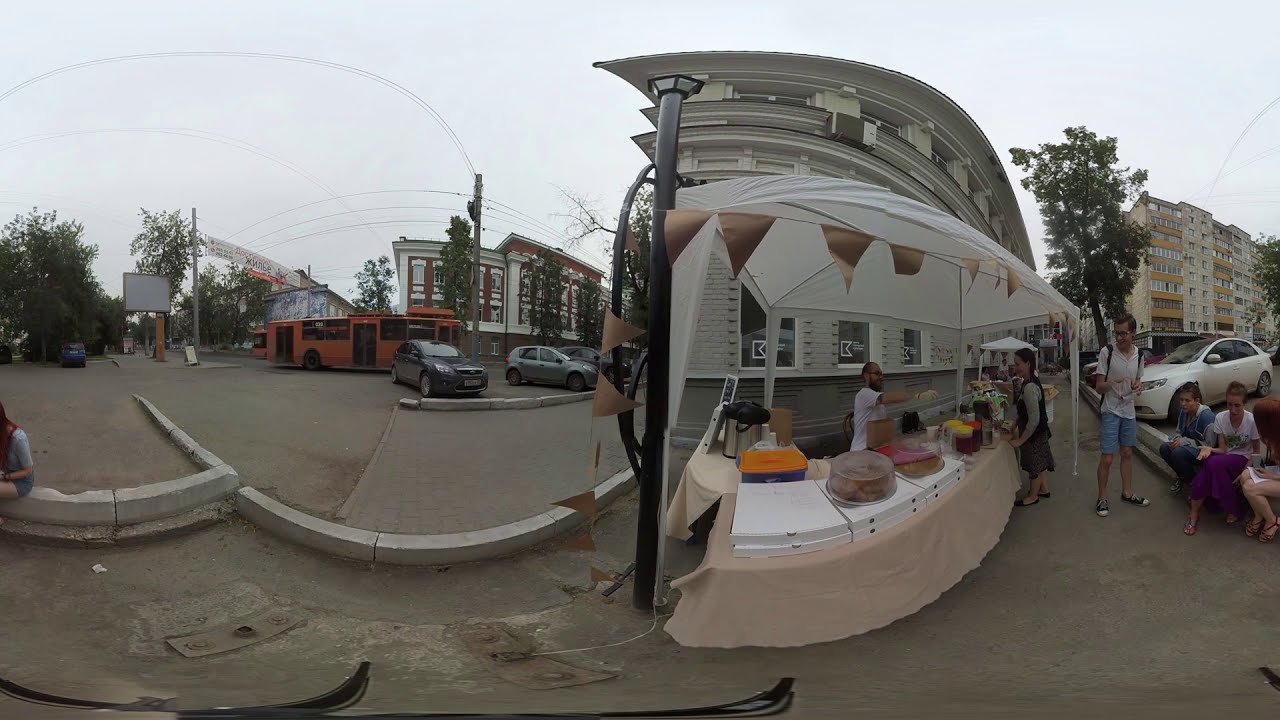The image captures a vibrant street scene featuring a food stall set up under a white tent adorned with brownish flags hanging down from its top. The tent houses a man in a white shirt and gloves, standing behind a long table covered with a light brown tablecloth. On the table, there are a variety of baked goods displayed in dome-shaped trays and numerous flat, white pizza boxes. In front of the stall, a woman in a black dress converses with the vendor while a small group of people lingers nearby on the sidewalk. 

To the left of the scene, an orange bus is driving by, and several cars are parked around the area, suggesting a bustling atmosphere. The background features a tall building that curves out of view, a network of telephone poles with numerous electricity lines, and some trees. The sky appears grayish and light blue, contributing to the overall mood of the setting, which feels warm and relaxed due to the casual attire of the people. On the far left, additional cars and an extended sidewalk can be seen, framing a dynamic and detailed urban landscape.